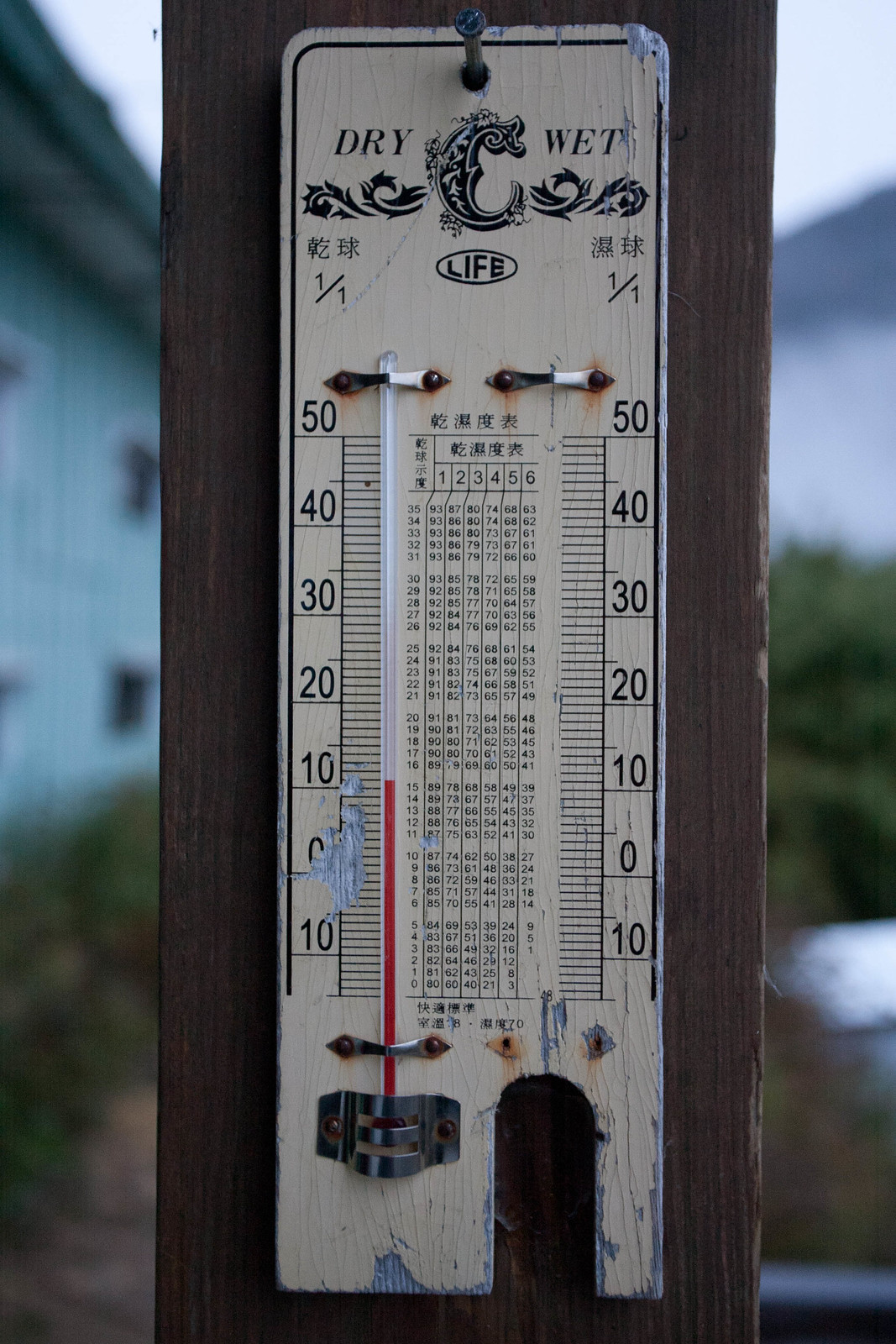The image features a weathered wooden thermometer stand, most likely from an Asian country, as suggested by the Asian script visible on the fixture. The stand is designed to hold two thermometers, but only the left one is present, containing red liquid typical of standard thermometers, and currently indicating 10 degrees. The scale on each side of the stand measures temperature from 10 to 50 degrees, although it is unclear whether this is in Celsius or Fahrenheit. 

The top of the stand is labeled with "dry" on the left and "wet" on the right, indicating the intended positions for the thermometers. Between the two thermometer slots is a central chart filled with numerous numbers and more Asian script beneath it. The wooden structure itself shows significant signs of wear and tear; chunks are missing, and the paint is notably worn off, especially towards the bottom, obscuring parts of the temperature scale. The entire piece appears to be nailed to another wooden post. In the background, there are hints of green-blue houses and some foliage, setting a rustic atmosphere around the somewhat decrepit thermometer stand.